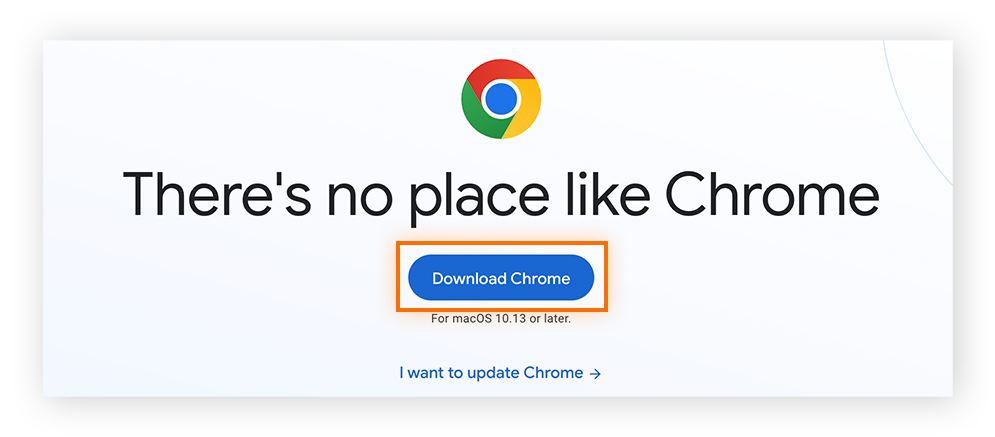This advertisement for Google Chrome, Google’s popular web browser, features a central tagline: "There's no place like Chrome," cleverly playing on the iconic phrase from The Wizard of Oz, "There's no place like home." Prominently displayed above this tagline is the recognizable Chrome logo, sporting its characteristic red, green, yellow, and blue colors.

Below the tagline, a highlighted blue button invites users to "Download Chrome." This button is clearly clickable, offering easy access for users looking to install the browser. Beneath this, text advises that the download is compatible with Mac OS 10.13 or later, indicating a specific target audience of Mac users.

At the bottom center of the advertisement, a blue hyperlink text reads, "I want to update Chrome," suggesting that the image may also be aimed at users who need to update their current version of the browser, or possibly indicating an issue with an existing installation. This line subtly implies a focus on ensuring users have the latest version of Chrome.

Additionally, a small blue line in the upper left-hand corner of the image, though its purpose is unclear, may be part of the UI design or another element of the visual layout.